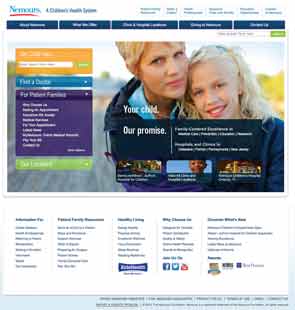Screenshot of the Nemours Children's Health System Webpage:

The webpage features an organized layout designed for ease of navigation, tailored to families seeking pediatric care. The top section includes navigation links such as "About Nemours," "What We Do," "News & Media," "Find a Nemours Location," "Giving to Nemours," and "Careers."

In the main section, there's a "Find a Doctor" search box, allowing users to locate doctors by location, specialty, or name. Additionally, there is a dedicated segment for "Top Pediatric Facilities," highlighting some of the leading healthcare facilities associated with Nemours.

The website prominently displays their commitment with messages like "Your Child, Our Promise," underscoring their dedication to children's health. The "Family-Centered Experience" section details their approach to providing care that involves the entire family.

"News and Events" offer updates on recent achievements and upcoming events relevant to the Nemours community. There are supporting sections for various links, including resources for patients and families, referring physicians, job seekers, and more. The "Patient Family Resources" section provides vital information and support for families.

The webpage also promotes "Healthy Living" and includes sections such as "Why Choose Us" and "Ways to Connect," which contain contact information, legal notices, privacy policies, and other essential links.

Overall, the design focuses on accessibility and offers comprehensive information aimed at assisting families in navigating pediatric healthcare services effectively.